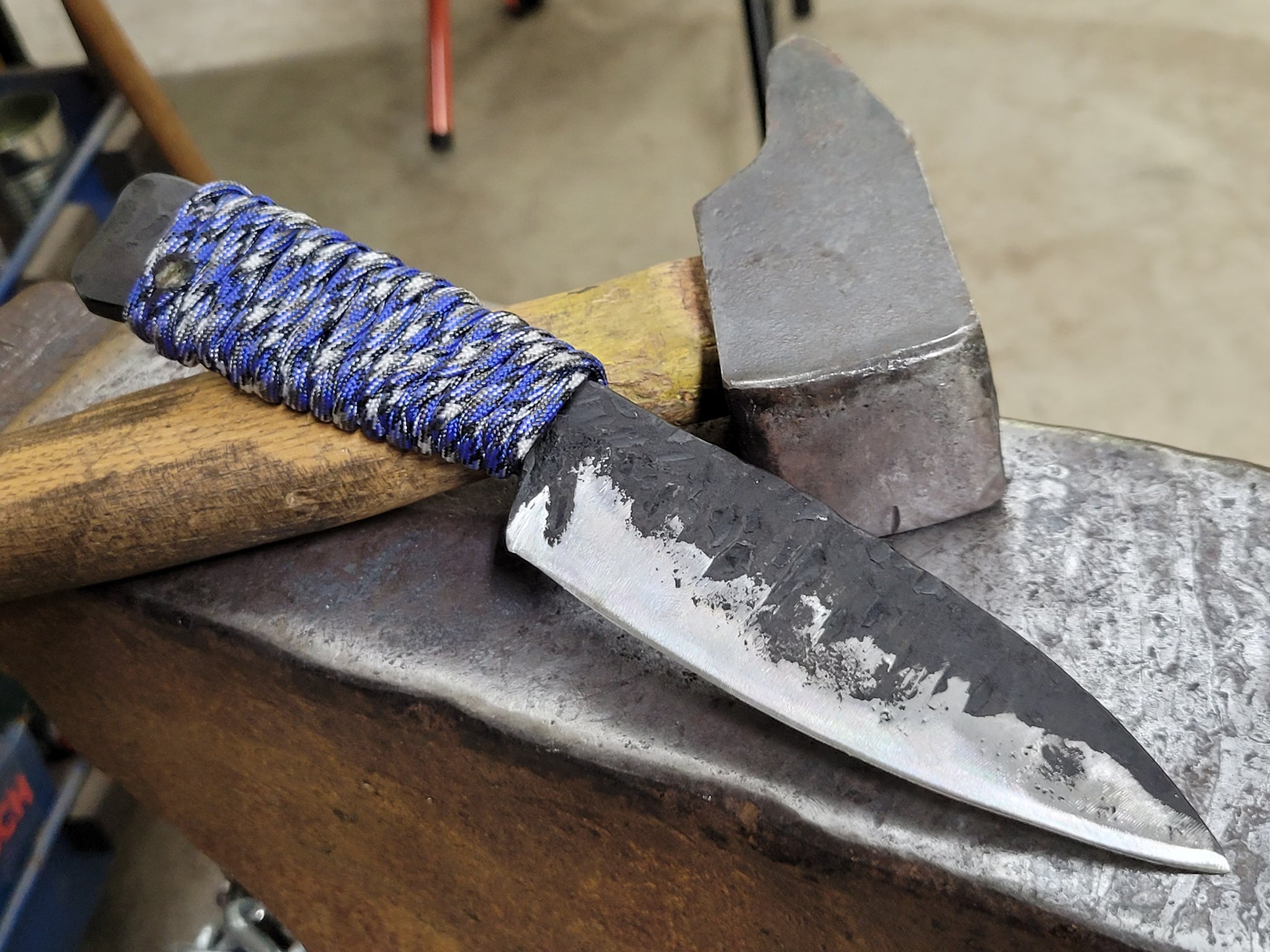The photograph captures a detailed, artistic display of a blacksmith's workbench positioned in a garage-like setting with a cement floor subtly blurred in the background. At the center of the image is an old-style blacksmith's anvil, exhibiting shades of gray, black, and rust. On top of this anvil lies a hammer with a wide, long wooden handle and a steel head featuring a square front and a rounded back. Alongside the hammer, centrally positioned, is an ornate knife. The knife boasts a distinctive blade with a black top and a silver cutting edge, complemented by a handle wrapped intricately with blue, black, and white rope, suggesting recent craftsmanship. The knife's and hammer's arrangement suggests a focus on the tools, emphasizing their importance and centrality to the blacksmith's work amidst the indistinct, board-like background.